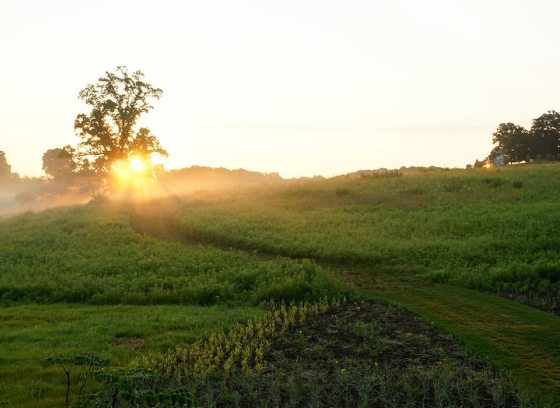This photograph captures a pastoral landscape dominated by a grassy field. A rough, mown path cuts through the center of the field, curving slightly and leading into the distance where it disappears amongst a stand of trees. The path, seemingly created by a tractor or a combine harvester, reveals patches of underlying soil where the grass growth is sparse. On the left side of the path stands a large, solitary tree, creating a focal point against the open sky.

To the right, near the top of the image, a small white house surrounded by a cluster of trees is visible, providing a hint of habitation in this rural setting. The sky above is a pale white, masking the time of day, though a setting or rising sun can be seen glowing faintly beyond the trees at the end of the path, casting a serene light over the scene. The overall mood suggests either early morning or late evening, adding a tranquil quality to the image. In the foreground, twigs and vines can be seen amidst the green vegetation, adding texture and depth to the idyllic countryside scene.